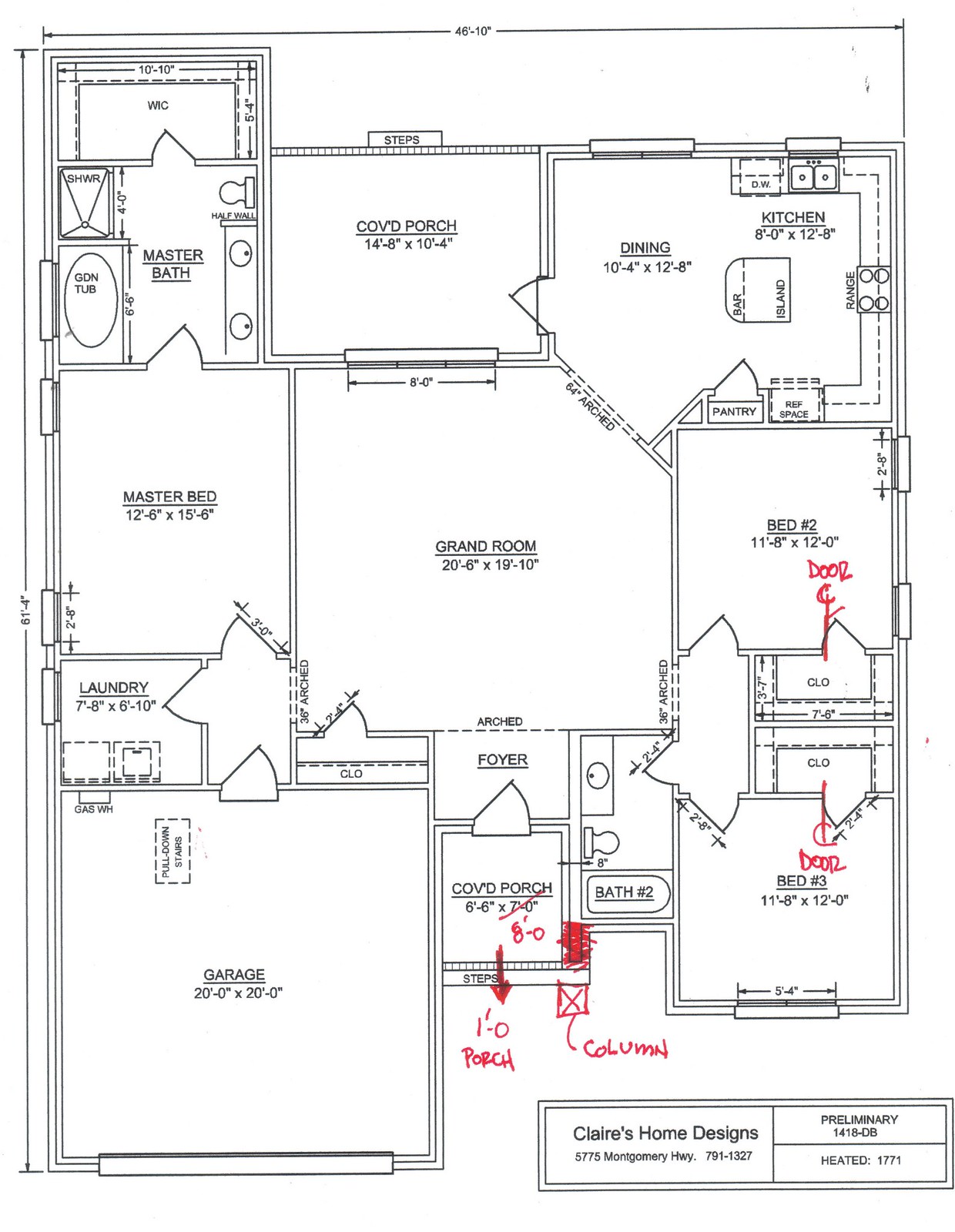This detailed blueprint, labeled "Claire's Home Designs," outlines a prototypical layout for a future house located at 5775 Montgomery Highway, with the preliminary design numbered 1418 DB. The heating area is noted to be 1771 sq. ft. 

Starting from the bottom and moving upwards, the floor plan showcases various rooms:

- **Garage**: The largest section of the blueprint, situated prominently.
- **Covered Porch**: A small area to the right of the garage.
- **Bathroom with Bathtub**: Adjacent to the covered porch.
- **Foyer**: Positioned to the left of the bathroom.
- **Bedroom 3**: Located next to the foyer.
- **Bedroom 2**: Positioned above Bedroom 3.
- **Grand Room**: The second largest space in the design, centrally located.
- **Laundry Room**: Sitting near the grand room.
- **Master Bedroom**: Alongside the master bathroom, situated towards the upper section of the plan.
- **Second Covered Porch**: Another small covered area.
- **Dining Room**: Small and adjacent to the kitchen.
- **Kitchen**: Includes a pantry, sinks, and stoves, adjacent to the dining room.

This preliminary design offers a comprehensive layout, detailing the spatial arrangement and function of each room to provide a vivid visualization of Claire's envisioned home.